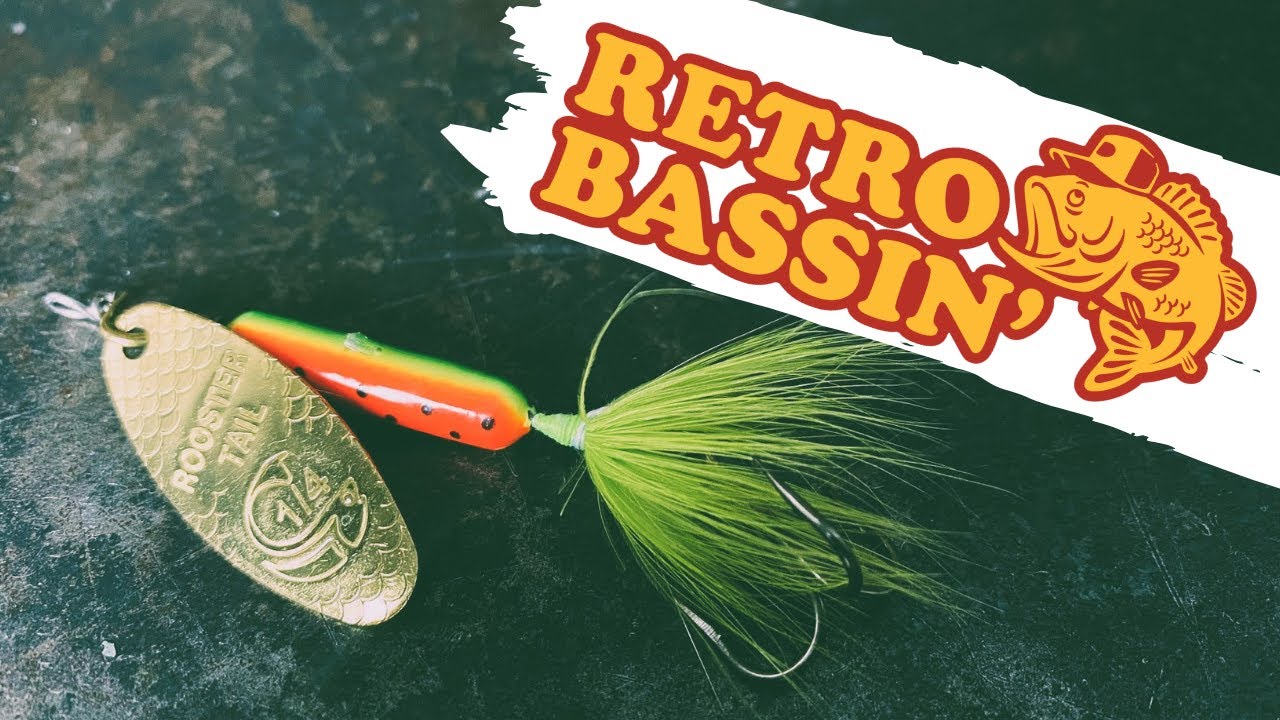The image appears to be an advertisement prominently featuring the words "Retro Bassin'" in bold yellow letters with a red outline, set against a white paint-like streak in the top left corner. To the right of this text is a cartoon depiction of a bass fish with its mouth open, sporting a baseball cap, following the same yellow with red border color scheme. Below and slightly to the left is a green surface, with multiple areas showing signs of scraped-away paint revealing a grey underneath. On this surface lies fishing equipment, including a silvery-gold, oval-shaped lure, embossed with the words "Rooster Tail" and an engraving of a fish. Adjacent to this is a vividly colored bait, featuring numerous fluorescent green strands, a bright orange section with a yellow stripe, and a cylindrical green piece, all connected to hooks. The overall setup suggests a detailed and vibrant fishing-themed advertisement or poster.